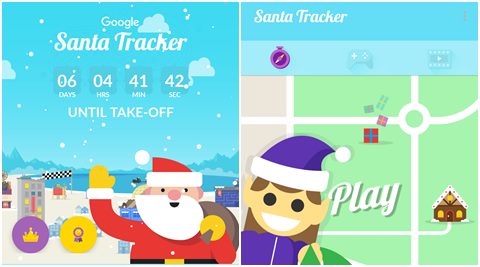This image is a screenshot from the Google Santa Tracker displayed on a desktop interface. The screen is evenly split into two halves, with a clean white outline dividing them.

On the left side, the background features a gradient blue sky transitioning from a deep sky blue to a lighter shade towards the bottom. Overlapping the sky are dark blue mountains capped with snow and fluffy white clouds. At the top, white text reads "Google Santa Tracker," followed by a countdown in smaller white lettering stating "Six days, four hours, 41 minutes, 42 seconds until takeoff."

Below this text, there is a sequence of graphical elements: a purple circle with a golden crown inside, directly to the right is a golden circle with a purple ribbon medal, and further to the right, Santa Claus appears. Santa sports his traditional attire— a red and white cap and suit, a big white beard, and he waves with one hand while holding a sack of toys in his other hand. Behind Santa, there is a checkered finish line with his reindeer positioned beside it, and the ground is covered with snow. Snow-capped buildings form the backdrop.

The right side of the screen is segmented into various interactive elements. At the top, the background is blue with "Santa Tracker" written in white letters. Below it, there is a purple stopwatch icon. Moving right, there are two grayed-out icons: a game controller and a play button, reminiscent of a movie play icon. Below these elements, a simplified map resembling Google Maps is displayed with a green background and white road markings. A gingerbread house is prominently marked on the map. To the left of this map stands an elf dressed in purple attire.